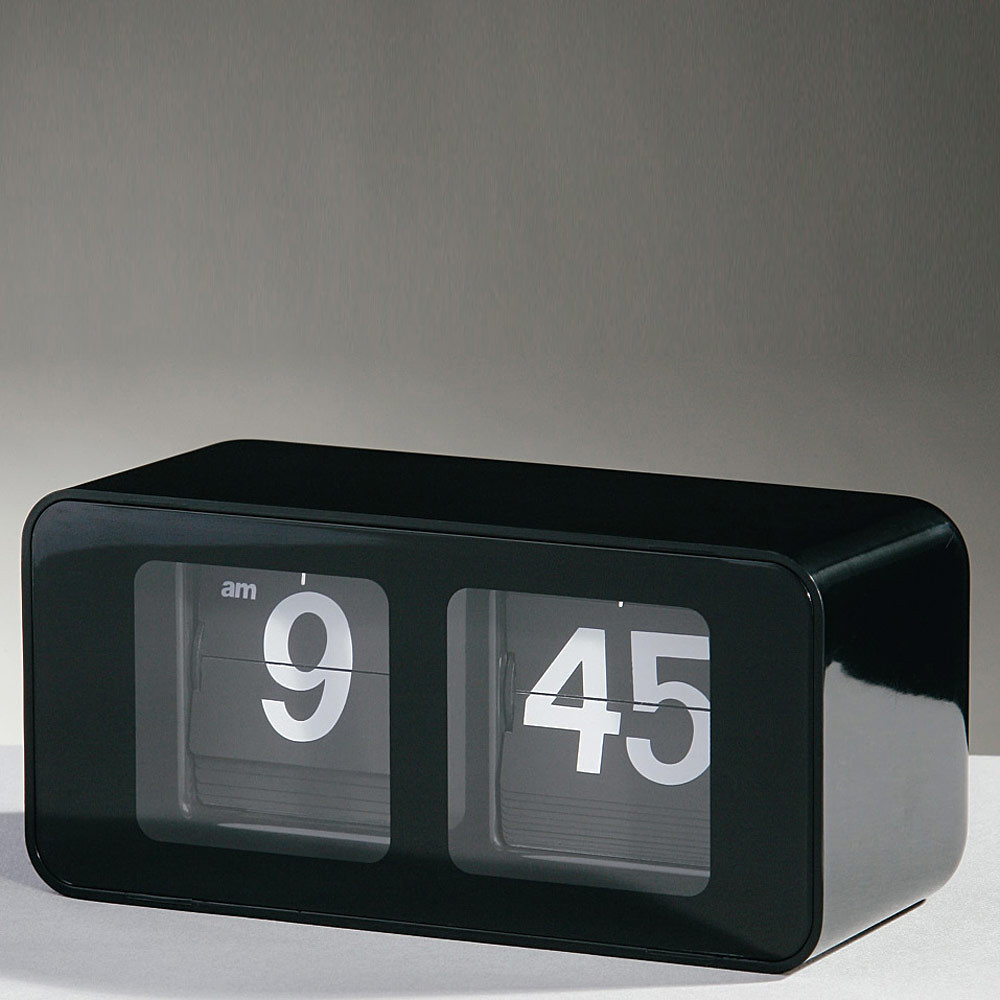The image features a sleek, modern alarm clock resting on a white table against a grey background. The alarm clock is designed in the style of a classic flip clock but with a contemporary twist. It is a black, rectangular prism with smoothly rounded corners, boasting a glossy finish that suggests a composition of either plastic, metal, or glass. The front of the alarm clock has two square windows, each with rounded corners. In the left window, the clock displays the number '9' along with 'AM', while the right window shows '45', indicating the time is 9:45 AM. The numbers and labels appear on flipping cards, reminiscent of vintage flip clocks, adding a nostalgic yet modern touch to the device.